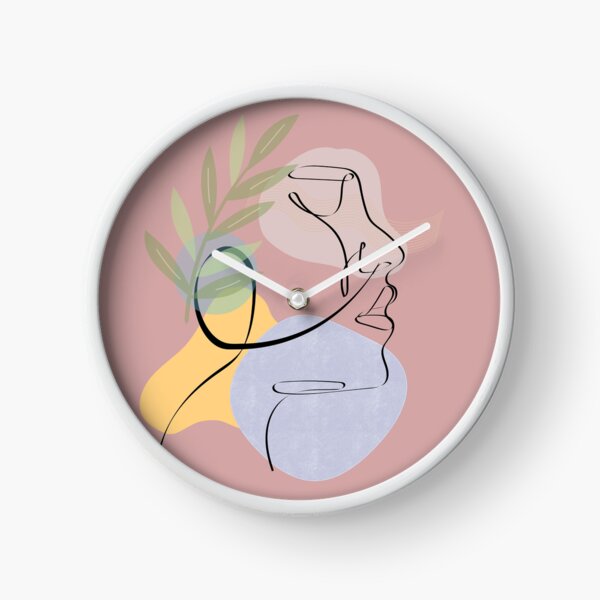The image depicts a stylish, modern analog clock with a minimalist aesthetic. The clock's face is circular with a thin white border, and the background is a striking rose-pink color. At the center of the clock are abstract elements: an outline of a woman's face, featuring a nose, mouth, chin, and a partial eye, rendered in simple lines. To the left of this face, there's a depiction of a green plant with varying shades of green leaves. Additionally, there is a blue rounded cube shape and a golden yellow freeform curved shape scattered across the face, adding to the abstract artistry. The clock lacks numerical markers, relying solely on two white hands for time-telling, which suggests it is approximately 10 minutes past 10 o'clock. The clock rests against a white background, enhancing its minimalist and modern appeal.